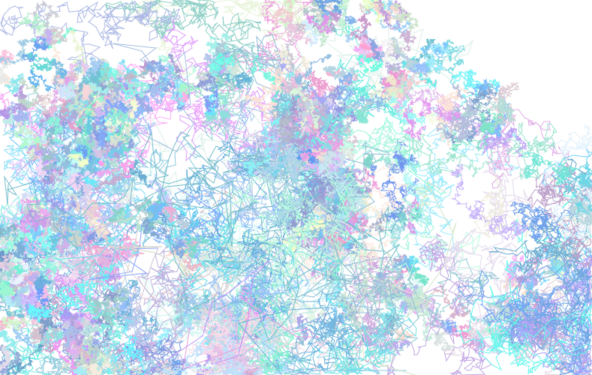This abstract painting, set on a white canvas, features an intricate mix of interconnected lines, squiggles, and splotches that evoke a sense of modern, almost chaotic art. Predominantly, the palette ranges from turquoise and dark blue to various shades of purple, lilac, and dark pink, with occasional touches of greenish-blue. Although the painting is filled with vibrant colors, white spaces, particularly in the upper right corner, provide striking contrast, and other patches of white shine intermittently throughout. This composition, reminiscent of a pastel-tone Jackson Pollock, presents an array of colors that blend together in some places while standing out distinctly in others, creating a dynamic and textured visual experience.